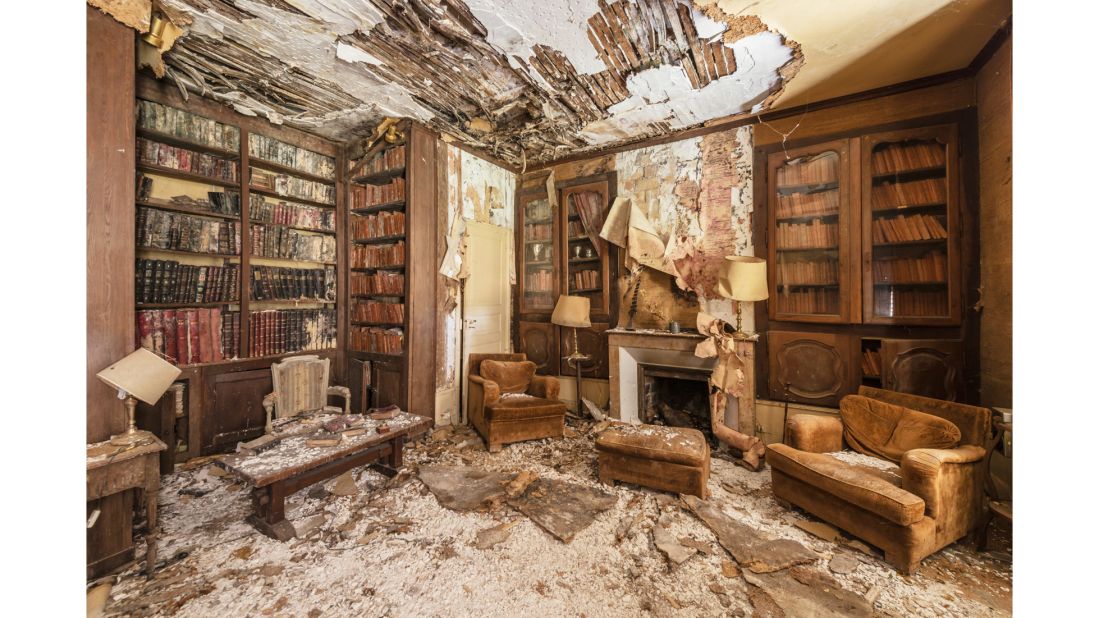The photograph captures a haunting scene inside an abandoned library room, likely within a house or building that has suffered significant damage. The ceiling is severely dilapidated, with large sections collapsed and exposing wooden beams. The remnants of the ceiling, including drywall and debris, litter the floor and furniture, creating a stark white mess amidst the prevalent browns of the space. 

In the center of the image stands a fireplace flanked by tall, wooden bookcases filled with books that reach up to the broken ceiling. To the left of the fireplace, a large wooden desk sits with an armchair beside it. Two velvet-style club chairs with a matching ottoman are positioned in front of the fireplace. Another towering bookcase and a smaller one nearby are equally stuffed with books. 

The room shows signs of severe water damage, with peeling wallpaper and sagging, rotted ceiling material. A lampshade teeters half-off a lamp, and the floor is almost entirely obscured by debris. This once serene reading room now teeters on the edge of ruin, its contents untouched and gradually succumbing to the forces of time and decay.